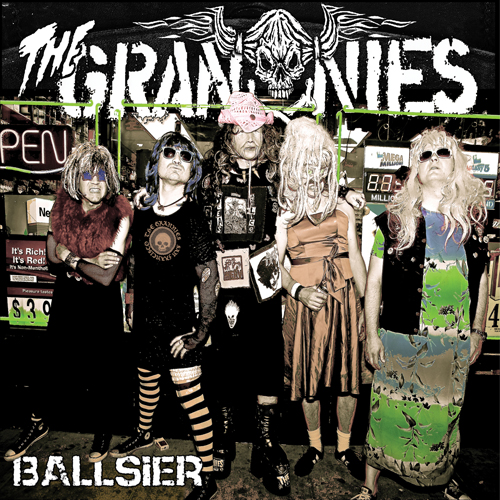This vertical rectangular image appears to be a band photo featuring five individuals dressed in eclectic and theatrical attire, suggestive of a punk rock drag ensemble. Set against a dark background that might be a gas station or storefront, the name of the band, "The Grannies," is displayed prominently at the top within a logo featuring a skull with wings. Below the emblem, the band members, who are all dressed to impersonate old ladies, stand out vividly. They sport attire such as white wigs, thrift store dresses, a fur shawl, and fishnet gloves. One of the members wears black and white striped leggings paired with a black t-shirt dress adorned with a skull, while another sports a pink cowboy hat and a heavy metal t-shirt. Converse All-Star tennis shoes and multicolored dresses enhance their eccentric look. At the bottom left of the image, the word "Ballsier" is visible, suggesting this is likely an album cover. The overall vibe is deliberately strange and visually striking, aiming to capture attention through a mix of humor and punk rock defiance.